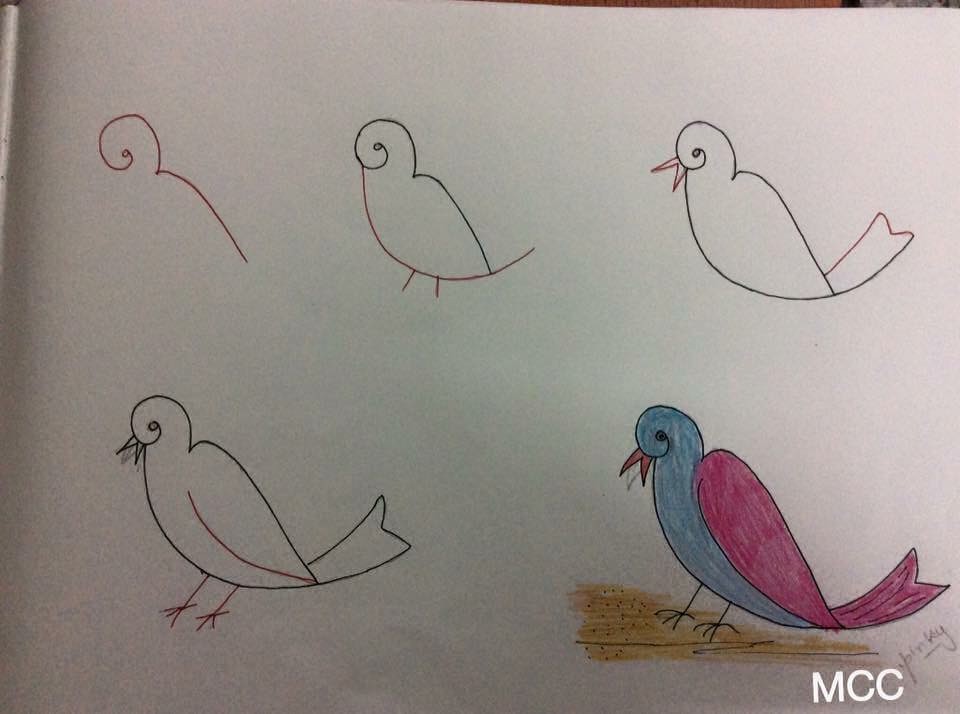In this close-up photograph of a drawing on a large piece of white drawing paper, a detailed step-by-step process for drawing a bird is illustrated through five sequential images. Each small picture captures a distinct phase of the bird's creation.

The first image starts with a curled line resembling a question mark drawn in red, forming the bird's back and head outline. Moving to the second image, the bird's back remains, now black, and a new line for the belly appears, along with the transition of the initial curly queue into black. By the third image, additional lines for the beak and tail are added, both in red, forming twin triangles at the top of the back for the beak, and a triangular tail. 

The fourth image extends the details by incorporating lines for the bird's feet and a partially drawn wing. Finally, the fifth image displays the fully drawn and colored bird. Its plumage features a blue breast and head, with a hot pink wing and tail, and an orange beak. The bird stands on a light brown splotch that represents soil, and it has black legs.

Artistically, the creator signs their name "Pinky" in pencil on the drawing, and a watermark reading "MCC" is superimposed in white text on the right-hand side.

This detailed progression not only showcases the technical steps of drawing a bird but also highlights the transformation from simple lines to a vibrant, fully realized illustration.